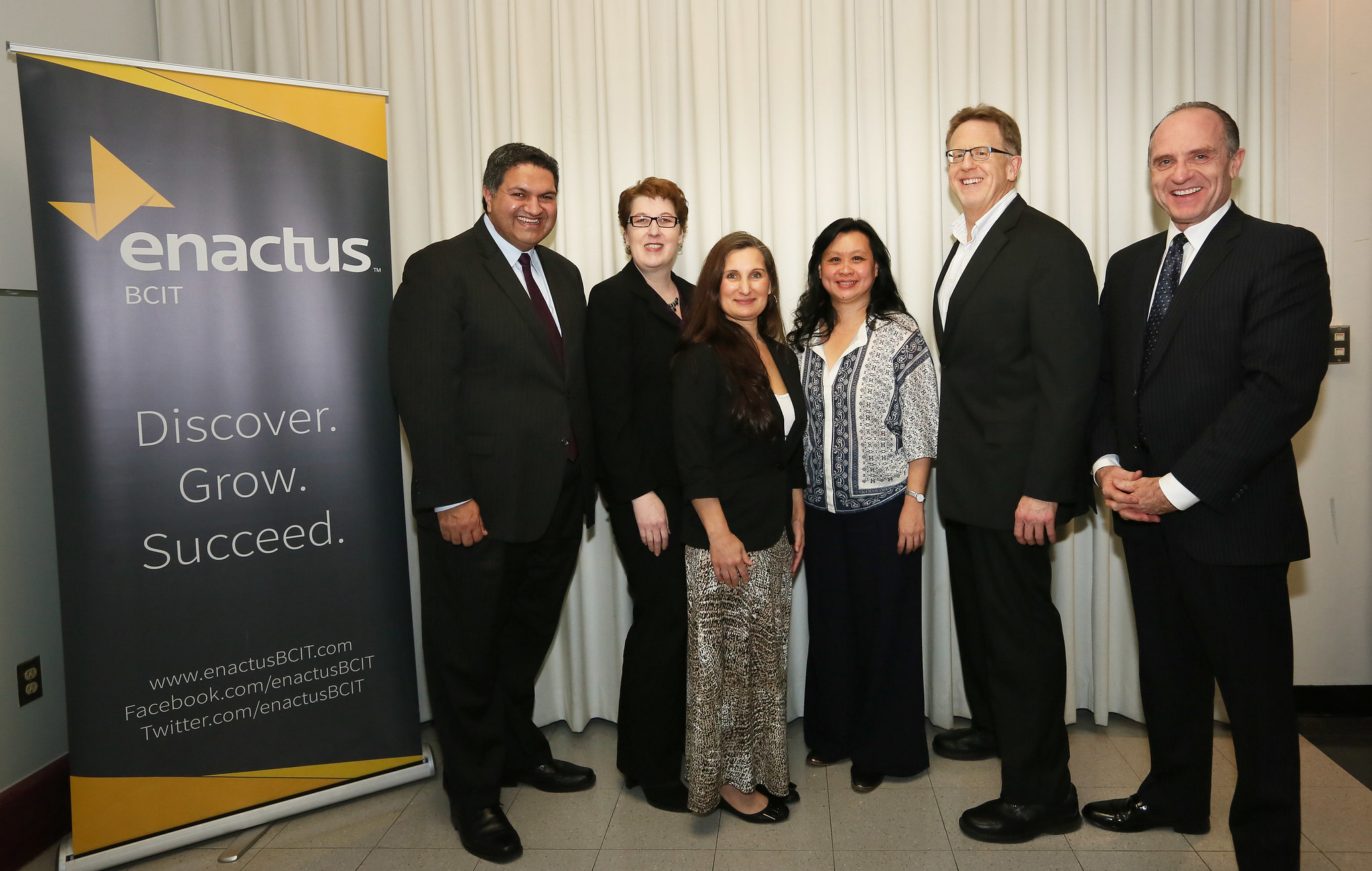This image captures a group of six individuals, likely attendees or speakers at a conference, standing in a line against a large white curtain. Behind them, a white wall with a few light switches can be partially seen. The group stands beside a stand-up banner prominently displaying the logo and branding for Enactus BCIT. The banner has a yellow top and bottom section with a predominantly black center, featuring the text: "Enactus BCIT Discover Grow Succeed," along with the website www.enactusbcit.com, and social media handles for Facebook and Twitter.

From left to right, the first person is a heavyset man dressed in a black suit with a white dress shirt and a tie. The second to fourth individuals are women with varied attire. The first woman is dressed in an all-black pantsuit, the second woman sports a leopard print skirt paired with a white t-shirt and topped with a black overcoat, and the third woman wears wide-legged black dress pants with a black and white button-up shirt. On the right, there are two men in black suits and white dress shirts; notably, the second-to-last man has a more casual look, omitting a tie and leaving his top button unfastened.